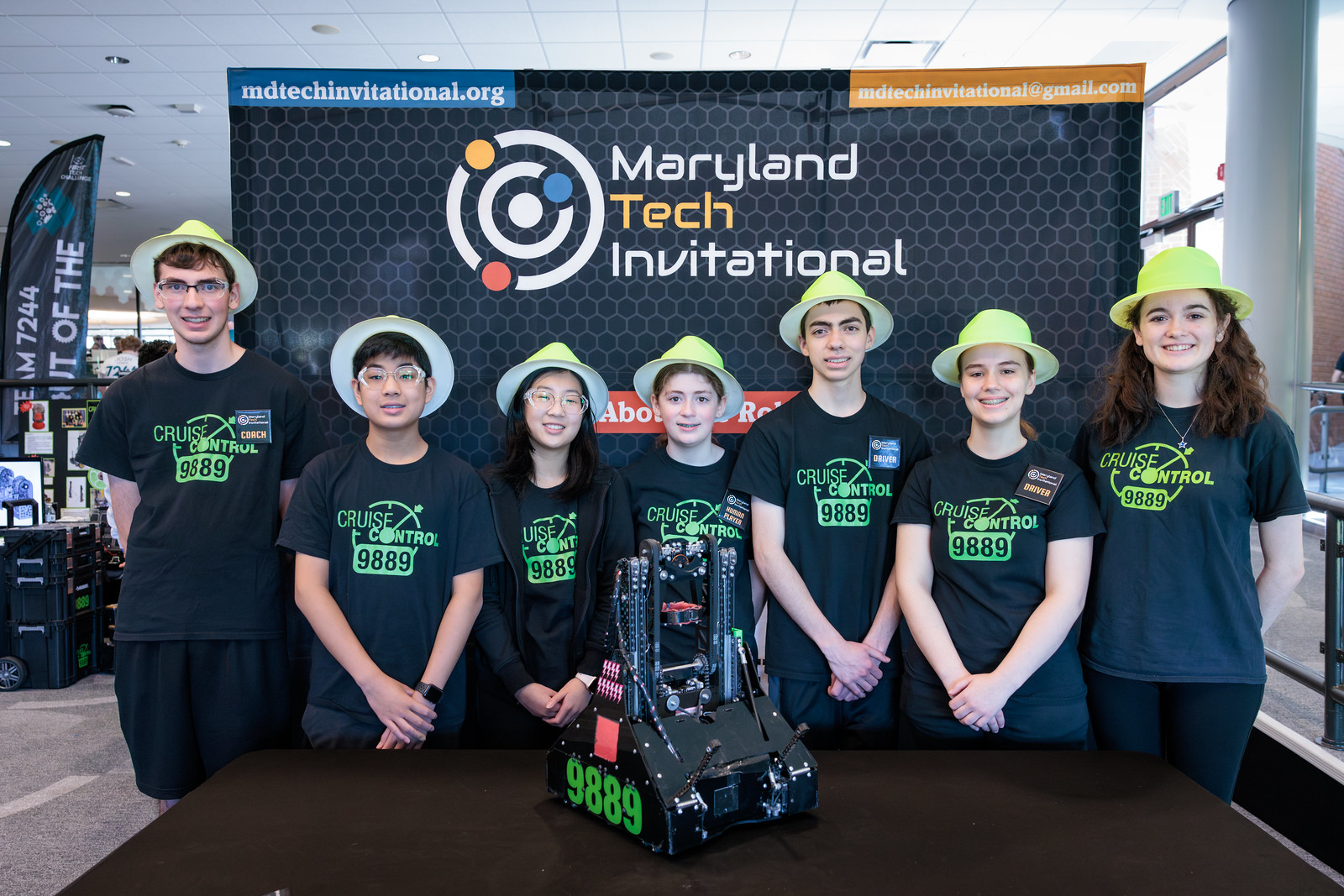In a vibrant indoor setting of a large conference room, a line of young boys and girls proudly stand behind a brown table, showcasing a sophisticated black robot machine they likely built themselves. The room, adorned with white ceiling columns and various displays and stands in the background, is bustling with presentations and booths, indicating an energetic tech conference. Prominently above them, a black banner reads "Maryland Tech Invitational," flanked by "mdtechinvitational.org" at the top left and "mdtechinvitational@gmail.com" at the top right. The left side of the banner features a target-like icon with concentric circles in yellow, red, and blue.

Each participant is dressed in a matching black t-shirt emblazoned with a green stopwatch design and the text "Cruise Control 9889." They also sport green hats, further unifying their team appearance. Three of the young people are distinguished by square badges that read "Driver." 

From left to right, the group includes a tall young man with glasses and brown hair, a shorter boy with black hair, a girl with long dark hair and glasses, a girl with short brown hair, a boy with very short brown hair, a girl with her light brown hair pulled back into a ponytail, and another girl with loose, curly brown hair. Together, they represent a coordinated and enthusiastic team, evidently proud of their technological creation and the collaborative effort it signifies.